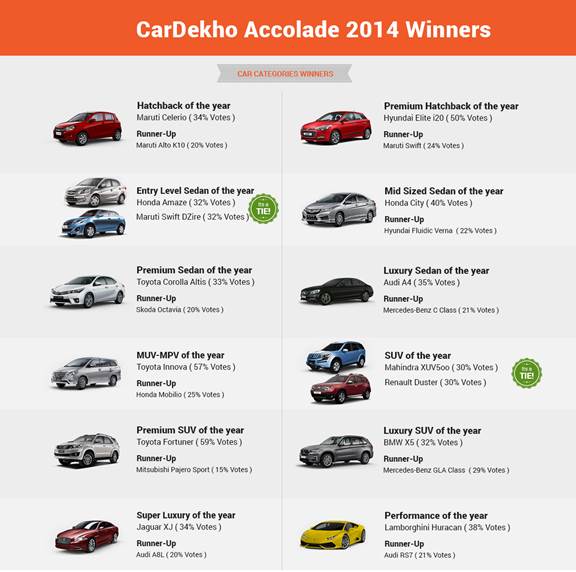**CarDekho Accolade 2014 Winners**

*An orange band at the top in white font reads: "CarDekho Accolade 2014 Winners." Below it, in two columns, there are six rows of award-winning cars, making a total of twelve cars. Beneath the "Accolade" banner, on a gray ribbon with orange font, it states: "Car Category Winners."*

**Hatchback of the Year:**
- **Winner**: Maruti Celerio with 34% of the votes
- **Runner-Up**: Maruti Alto K10 with 20% of the votes
- (Top left section)

**Premium Hatchback of the Year:**
- **Winner**: Hyundai Elite i20 with 50% of the votes
- **Runner-Up**: Maruti Swift with 24% of the votes
- (Top right section)

**Entry-Level Sedan of the Year:**
- **Winner**: Honda Amaze with 32% of the votes
- **Runner-Up**: Maruti Swift Dzire with 32% of the votes
- (Middle section)

*Each section showcases a sample car image pertaining to the winner and runner-up. Additionally, there appears to be a green award emblem in one of the sections, but its details are not clearly visible.*